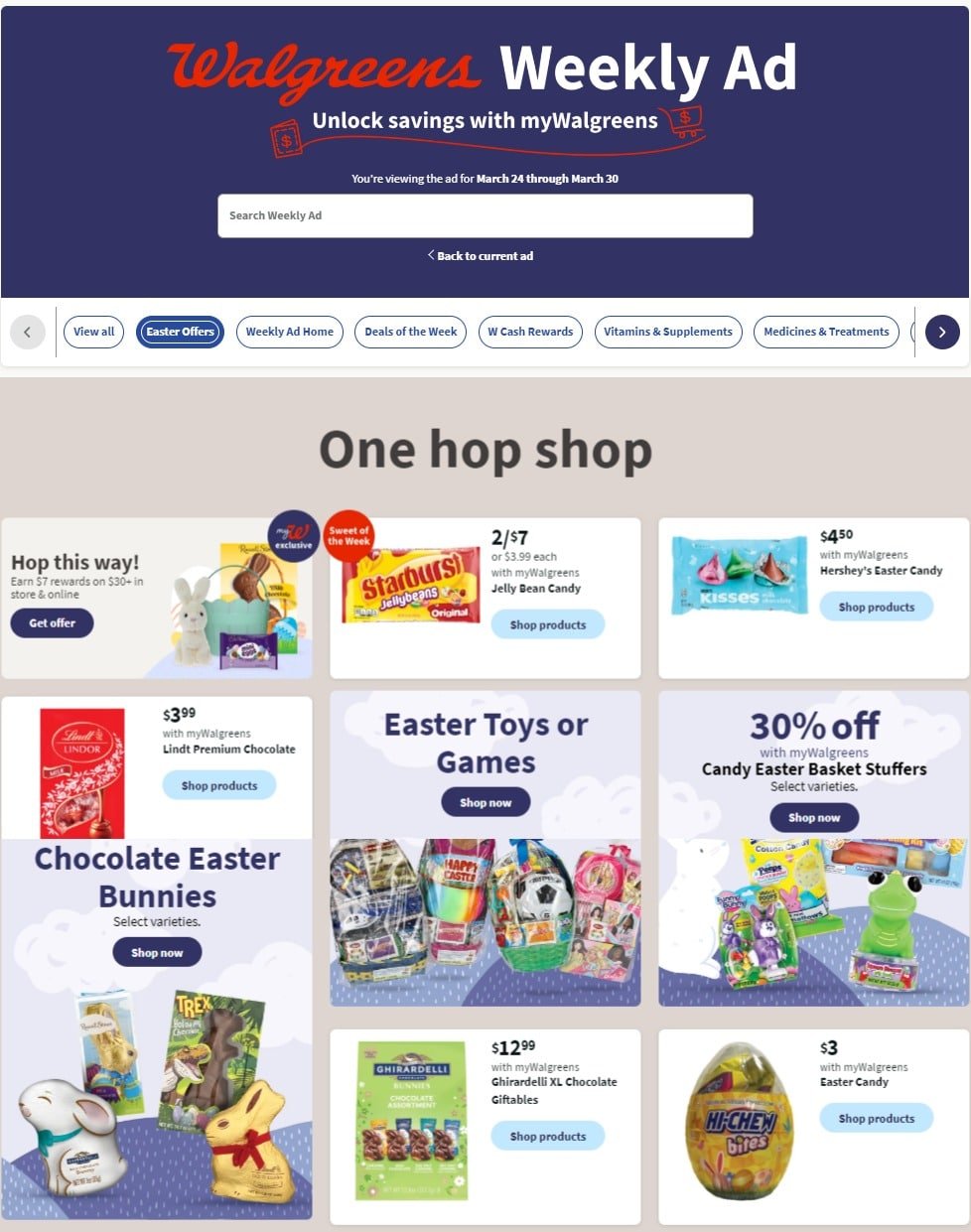In the image, we see a screenshot of the Walgreens app, prominently displaying the "Walgreens Weekly Ad" at the top center. The word "Walgreens" is in red, while "Weekly Ad" is in white. Below this, there's a section encouraging users to "Unlock Savings with myWalgreens," flanked by a shopping cart icon on the right and a money bag icon on the left. Immediately beneath this message is a search bar labeled "Search Weekly Ad" set against a white background.

Moving to the central portion of the image, the words "One Hop Shop" are boldly written in black on a gray background. Surrounding this header, multiple boxed sections showcase various products. In the top left box, there's a promotional text that reads "Hop this way, earn $7 on $30+ in-store/online" alongside an image featuring Easter-themed eggs. To the right of this box, there is a box displaying "Starburst Jelly Beans." 

In the middle section beneath this, the focus shifts to "Hershey Easter Candy," while to the right, another box highlights "Easter Toys or Games." At the bottom right corner, a section indicates "30% off" with a focus on Easter candy. To the left of this, there's an image of egg-shaped candies labeled "Bites." Finally, at the bottom left of the image, there's a feature on "Chocolate Easter Bunnies," illustrated with four chocolate bunny images.